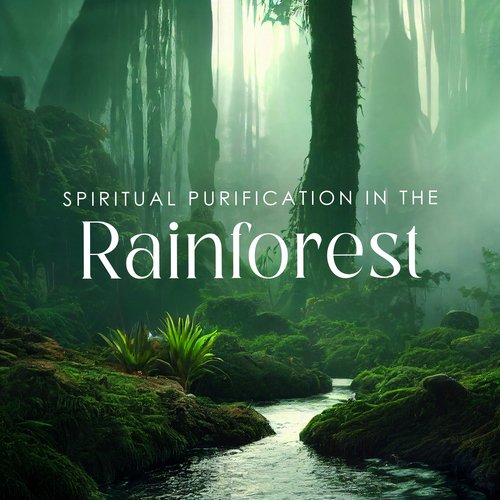The image portrays a lush rainforest scene, bustling with greenery and a diverse array of trees and vines. Soft green light filters down from above, bathing the forest floor in a serene glow. Green moss carpets the banks of a rushing creek, adding to the vibrant, natural ambiance. Overlaid on this picturesque view, in white text with a mix of sans-serif and serif fonts, is the phrase "Spiritual Purification in the Rainforest." This seems to signify a program or activity centered around cleansing the spirit amidst the tranquil beauty of the rainforest, possibly serving as an advertisement for such an experience.